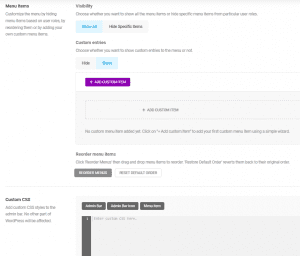The image depicts a very blurry screenshot against a white background. Starting from the top left, there are two words in bold black print, likely saying "Menu," though it is not entirely clear. Below that, four lines of light gray text are visible but too blurry to read. Moving to the right, beneath a light gray border, the word "Visibility" appears in bold black text. The following line includes additional text, but most of it is illegible, except for the partial phrase "choose whether you want to."

Beneath this line are two buttons: a light blue button with two words in dark blue text, and to its right, a white button with three words in black text. Continuing down, there are two more words in bold black text which are unreadable, followed by a line of gray text containing the phrase "choose whether you."

Further down are another set of buttons: on the left, a white button labeled "Hide," and to its right, a blue button with an illegible word. Below these buttons is a prominently placed purple button.